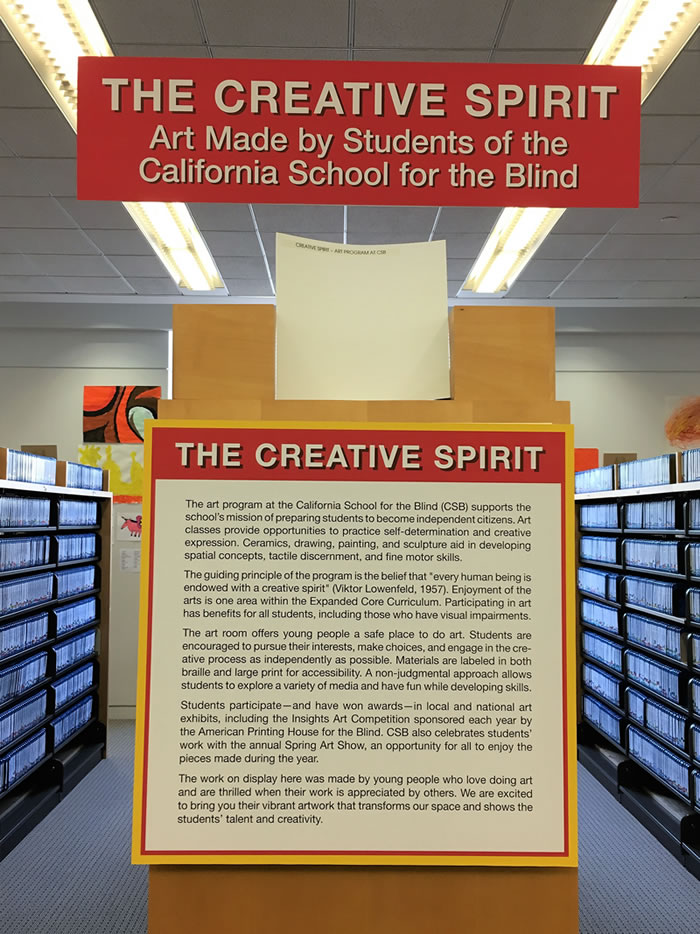In the picture, we see the interior of a library or classroom featuring a prominent display dedicated to an art program. At the top, a vibrant red poster with white lettering reads, "The Creative Spirit: Art Made by Students of the California School for the Blind." Below this header, the poster contains multiple paragraphs of text in black, with key points about the art program at the California School for the Blind (CSB), highlighting its mission to support students in becoming independent citizens and detailing the benefits of art classes like ceramics, drawing, painting, and sculpture in developing spatial concepts, tactile discernment, and fine motor skills. Surrounding the central display are shelves lined with blue objects, possibly books or files. The wall to the left of the display features a small drawing of a pink unicorn, while an abstract art piece in shades of orange, brown, and black hangs nearby. The room is well-lit with large fluorescent lights on the ceiling, adding a bright ambiance to the space.